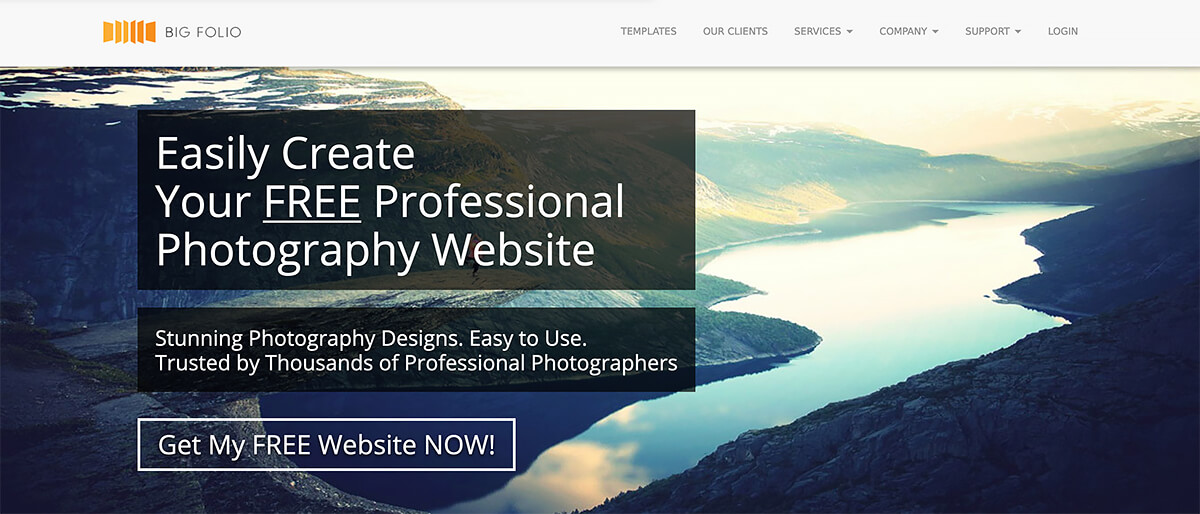This is a screenshot of the home page of a website named Bigfolio. At the top of the page, there is a gray navigation bar that features the website's orange logo on the left, followed by several navigation tabs to the right: "Templates," "Our Clients," "Services," "Company," "Support," and "Log In," each with dropdown menus where applicable.

Beneath the navigation bar, there is a horizontal photographic image that captures a serene river winding its way between two towering, mountainous banks. Snow-capped peaks can be seen in the background on both the left and right sides of the image. The colors of the photograph are primarily various shades of blue and green, contributing to a tranquil and picturesque scene.

Overlaying the photograph, there are three text boxes:
1. The topmost black box contains white text that reads, "Easily create your FREE professional photography website," with "FREE" in all caps and underlined.
2. The second black box below it states, "Stunning photography designs, easy to use, trusted by thousands of professional photographers."
3. The bottommost box is clear and contains white text within a pill-shaped button that says, "Get My Free Website Now," indicating it's a clickable call-to-action button.

This layout effectively combines visual appeal with clear calls-to-action and easy navigation, inviting professional photographers to explore and create their own websites using Bigfolio's services.